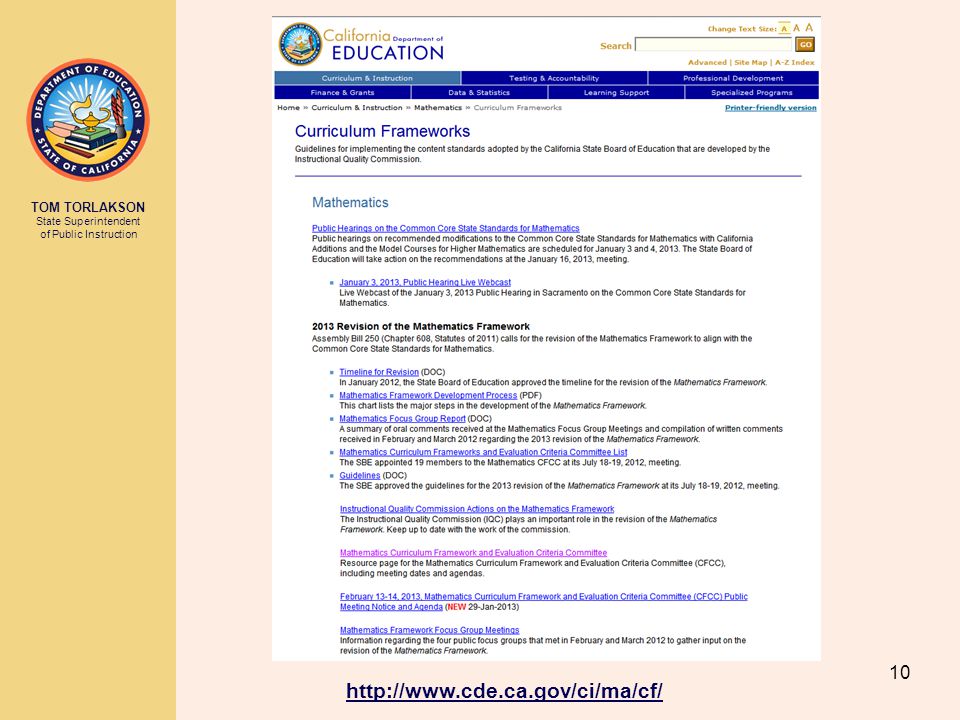The image showcases a webpage for the Department of Education in the State of California. Prominently featured is Tom Solaxson, the State Superintendent of Public Instruction. The content is dense with text, outlining various sections and information available on the webpage. At the top, key sections include Curriculum and Instruction, Testing and Accountability, Professional Development, Finance and Grants, Data and Statistics, Learning Support, and Specialized Programs. 

Additional text provides detailed information about the Curriculum Frameworks and Guidelines for implementing the Content Standards adopted by the California State Board of Education, developed by the Instructional Quality Commission. Specific to Mathematics, there are announcements about public hearings on recommended modifications to the Common Core State Standards for Mathematics with California Additions and the Model Courses for Higher Mathematics. These hearings are scheduled for January 3rd and 4th, 2013, and it's noted that the State Board of Education will take action on these recommendations during their meeting on January 16, 2013.